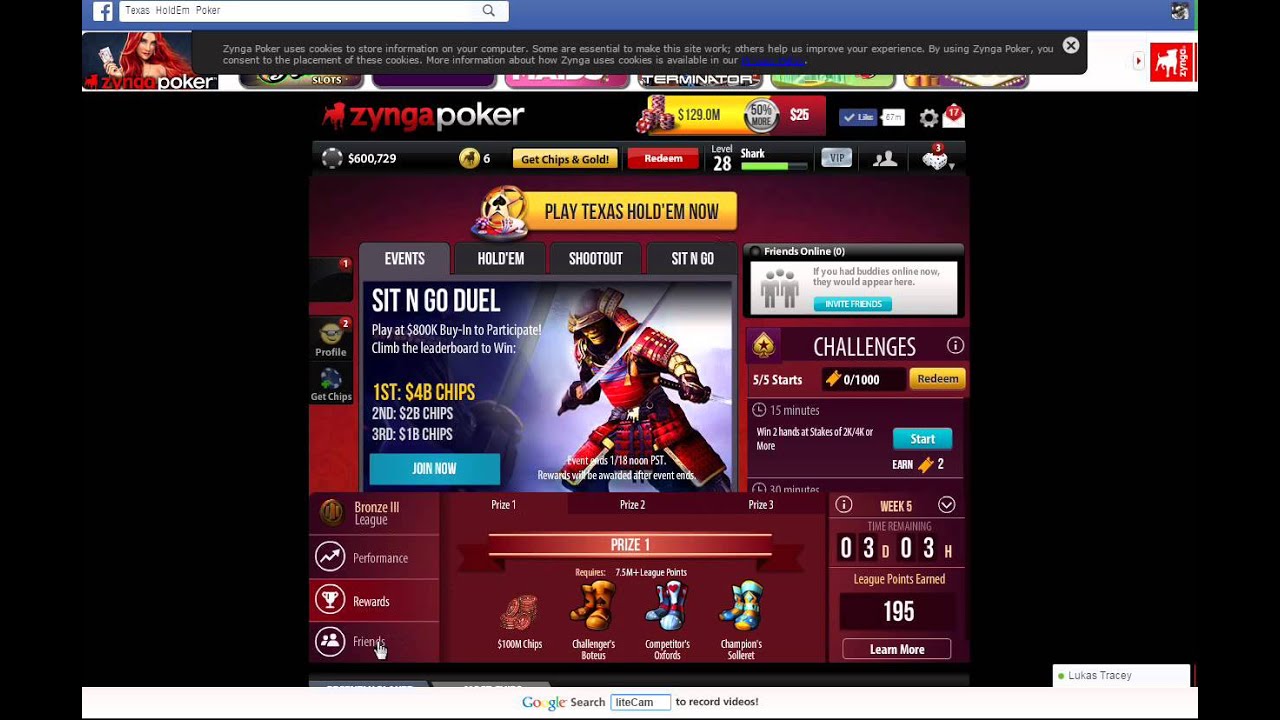The image is a screenshot of a web advertisement prominently featuring a Facebook banner at the top, characterized by its signature long, blue bar adorned with the white Facebook "F" logo. The user has performed a search for "Texas Hold'em poker," which has triggered the display of a Zynga Poker banner ad. 

Central to the advertisement is a vibrant, eye-catching graphic of a redhead woman with long hair, beside the recognizable white Zynga dog logo. A colorful pop-up box dominates the visual, heralding "Zynga Poker" with a vivid palette of yellows, reds, blues, and purples. The pop-up highlights an invitation to "Play Texas Hold'em Now" in a prominent yellow bar. Below this, there's an engaging depiction of a pirate clad in a red outfit, brandishing a sword, promoting a "Sit and Go Duel." The competitive rewards are also listed: first place stands to win 44 billion chips, second place offers 28 billion chips, and third place nets 1 billion chips.